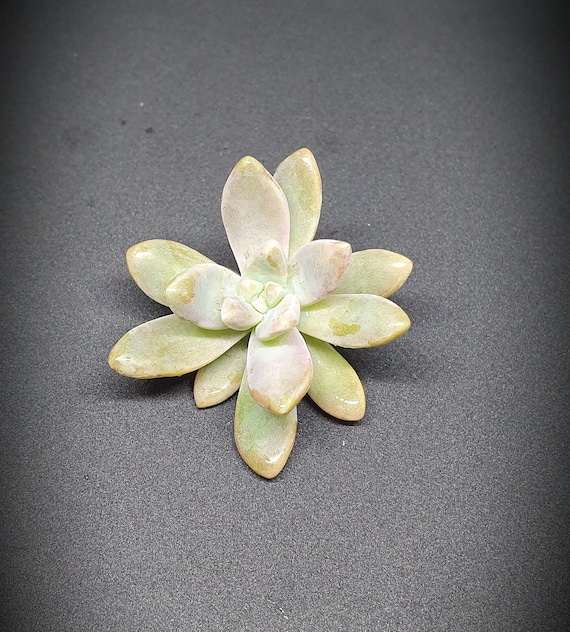The photograph depicts an elegantly crafted flower, likely resembling a lily or lotus, positioned on a charcoal gray, grainy surface. The flower appears to be made from a light green material, possibly pale jade, ceramics, or a glass-like substance, casting a soft shadow on the table. The petals, which radiate out from the center in a pointed, plus-like shape, transition from yellowish-green on the edges to white and pink closer to the center. The central area of the flower features smaller, delicate petals, signifying intricate craftsmanship. The edges of the image fade into a darker hue, highlighting the flower's delicate, waxy texture and creating a striking contrast with the gray background. This detailed object could be an ancient, delicate brooch or simply an exquisite display piece.